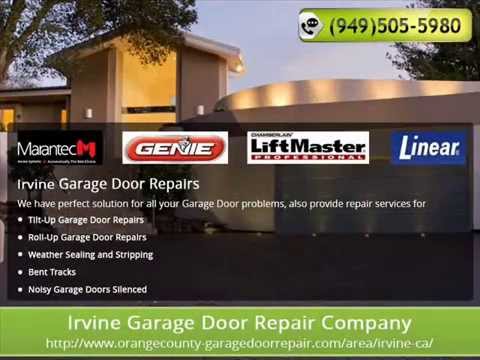This advertising image for a garage door repair company features a serene evening backdrop with a white house and a closed garage door. The sky is a rich, dark blue, indicative of the setting sun. On the upper right-hand side, there is a green box prominently displaying the company's phone number for easy access. Centrally, a translucent overlay contains logos of four notable brands: Marantec, Genie, LiftMaster, and Lanier. Below this, a bullet list highlights the services offered by "Irvine Garage Door Repairs," including tilt-up and roll-up garage door repairs, weather sealing and stripping, bed track maintenance, and solutions for reducing noisy garage doors.